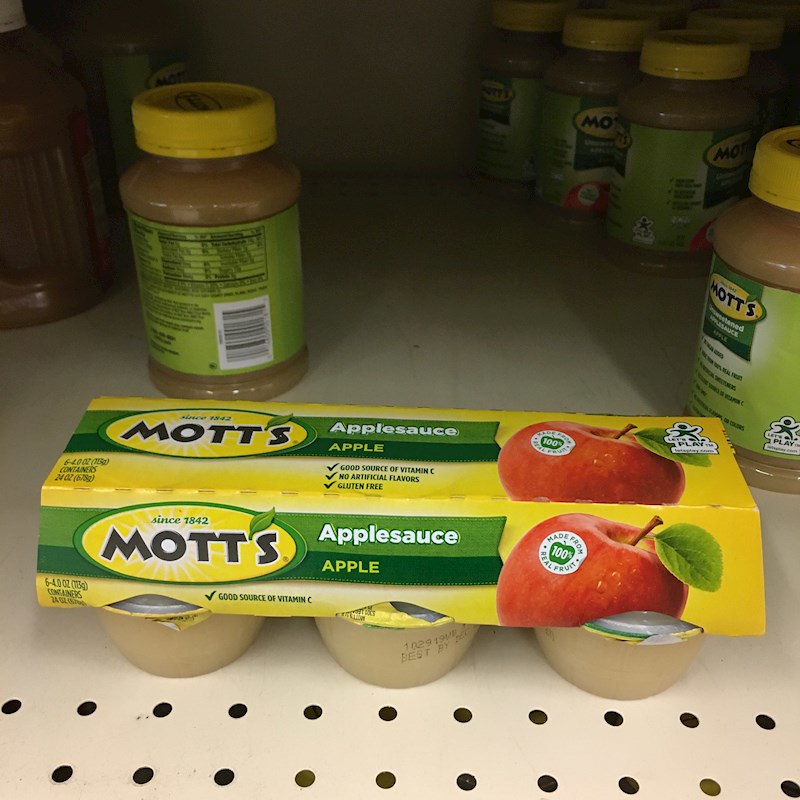The photograph captures a close-up of a bottom shelf in a grocery store, primarily featuring Mott's applesauce. The applesauce is prominently displayed in various forms: smaller plastic cups in an unopened six-pack and jars in the background. The six-pack, positioned in the foreground, has a bright yellow and green label with the Mott's logo in black letters on the left and a red apple on the right, emblazoned with a "100%" sticker. The plastic cups have their bottoms exposed, while the tops are covered by the vibrant packaging. The shelf itself is a tan industrial metal with sequential perforations along the front edge, and appears well-lit, in contrast to the darker background. Behind the six-pack, the shelf holds several jars of Mott's applesauce with green labels and yellow lids, including cinnamon apple and regular apple varieties. Additionally, there is a glimpse of vegetable juice on the left side of the image. The overall setting suggests a neatly organized grocery store aisle dedicated to shelf-stable products.